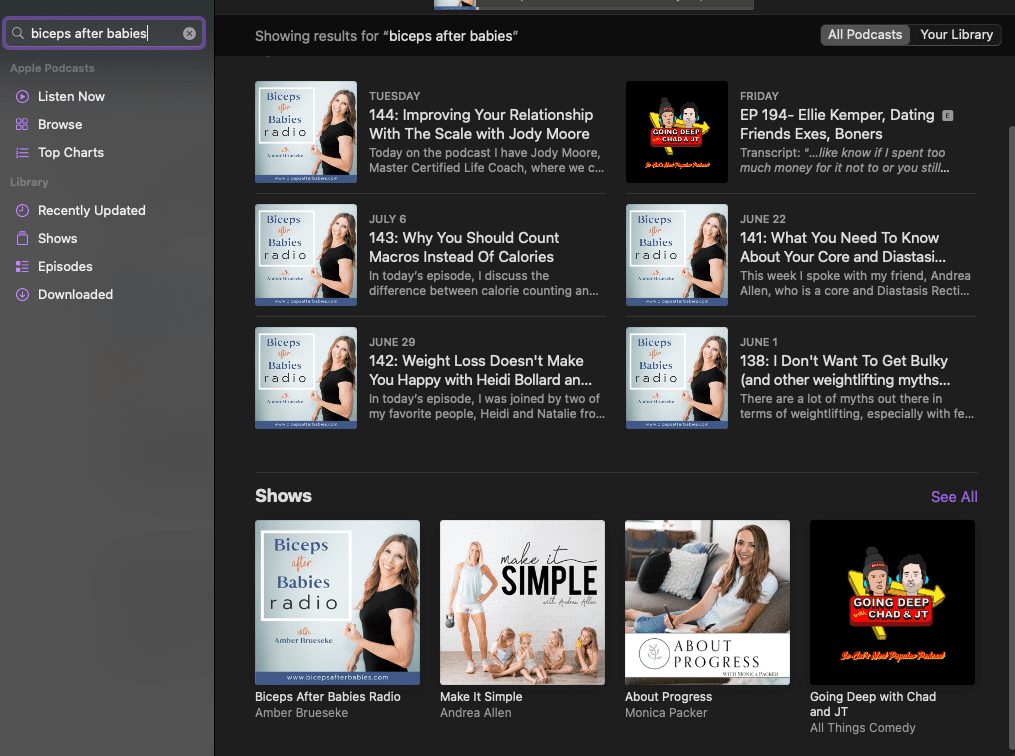This image showcases the search results for "Biceps After Babies" on a podcast service platform. The interface features a two-toned background: a light gray on the left and a dark, almost black, on the central and right portions. 

On the left side, a search bar in the top corner displays the query "biceps after babies." Below the search bar are navigation options including "Apple Podcasts," "Listen Now," "Browse," and "Top Charts." The library section underneath these options lists categories such as "Recently Updated," "Shows," "Episodes," and "Downloads."

In the middle section, the search results headline reads "Showing results for 'biceps after babies'." Two tabs are present: "All Podcasts" and "Library," with "All Podcasts" highlighted. The search results include:

- "Tuesday 144: Improving Your Relationship with the Scale" with Jodi Moore.
- "Friday, Episode 194: Ellie Kemper — Dating Friends, Exes, and Boners" marked as "Going Deep."
- "July 6th 143: Why You Shouldn't Count Macros Instead of Calories."
- "June 22nd 141: What You Need to Know About Your Core and Diastasis."
- "June 29th 142: Weight Loss Doesn't Make You Happy" with Heidi Bollard.
- "June 1st 138: I Don't Want to Get Bulky and Other Weightlifting Myths."

At the bottom of the results, various podcast shows are listed:
- "Biceps and Babies Radio."
- "Make It Simple" with Andrea Allen.
- "About Progress" with Monica Packer.
- "Going Deep" with Chad and JT, labeled under "All Things Comedy."

This detailed overview of the search results gives a comprehensive look at the content available related to "Biceps After Babies."